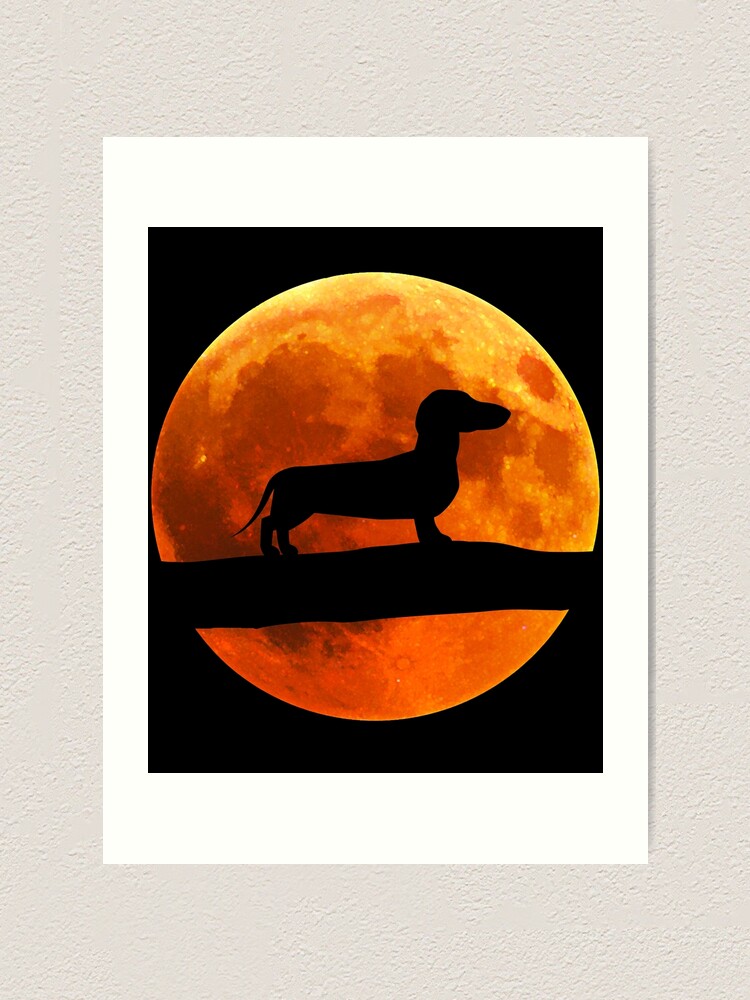The image is composed of three nested rectangles. The outermost and largest rectangle features a textured stucco wall in a light gray color. Inside this, a simple white rectangular border frames the central focus. The innermost rectangle is completely black, prominently showcasing an orangish-red, large, blood moon. The moon, which transitions from a deep, almost red-orange in the middle to a golden orange at the top, commands attention as the most striking feature of the image. Silhouetted against this vivid moon is a tree branch, situated about one-third down from the top. Above this branch, in the exact center of the image, is the profile silhouette of a dachshund, with its nose pointing to the right and its tail to the left. The sharp outline of the dog stands out against the glowing background, creating a captivating contrast that draws the viewer’s eye to the center of the scene.